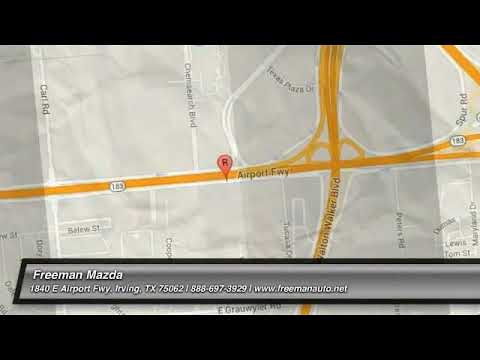The image is a detailed map depicting the location of Freeman Mazda at 1840 East Airport Freeway, Irving, Texas 75062. At the top and bottom, there are black bars; the bottom bar contains a gray section with white text providing the dealership's address, phone number (888-697-3929), and website (www.freemanauto.net). The central part of the image features a map with the Airport Freeway highlighted in yellow, stretching across the map. The freeway's name, "Airport Freeway," is written in white text running left to right and then top to bottom. A distinct red pin symbol, marked with an ‘R,’ indicates the exact location of Freeman Mazda on the freeway. Surrounding the freeway are various streets illustrated in different shades of gray, with their names labeled in white. A prominent white circle with the number ‘183’ in black is situated to the left of the red pin, further detailing the nearby roads. The overall map utilizes a top-down perspective, showcasing the freeway, surrounding streets, and landmarks, aiding in navigation to Freeman Mazda without missing the dealership.